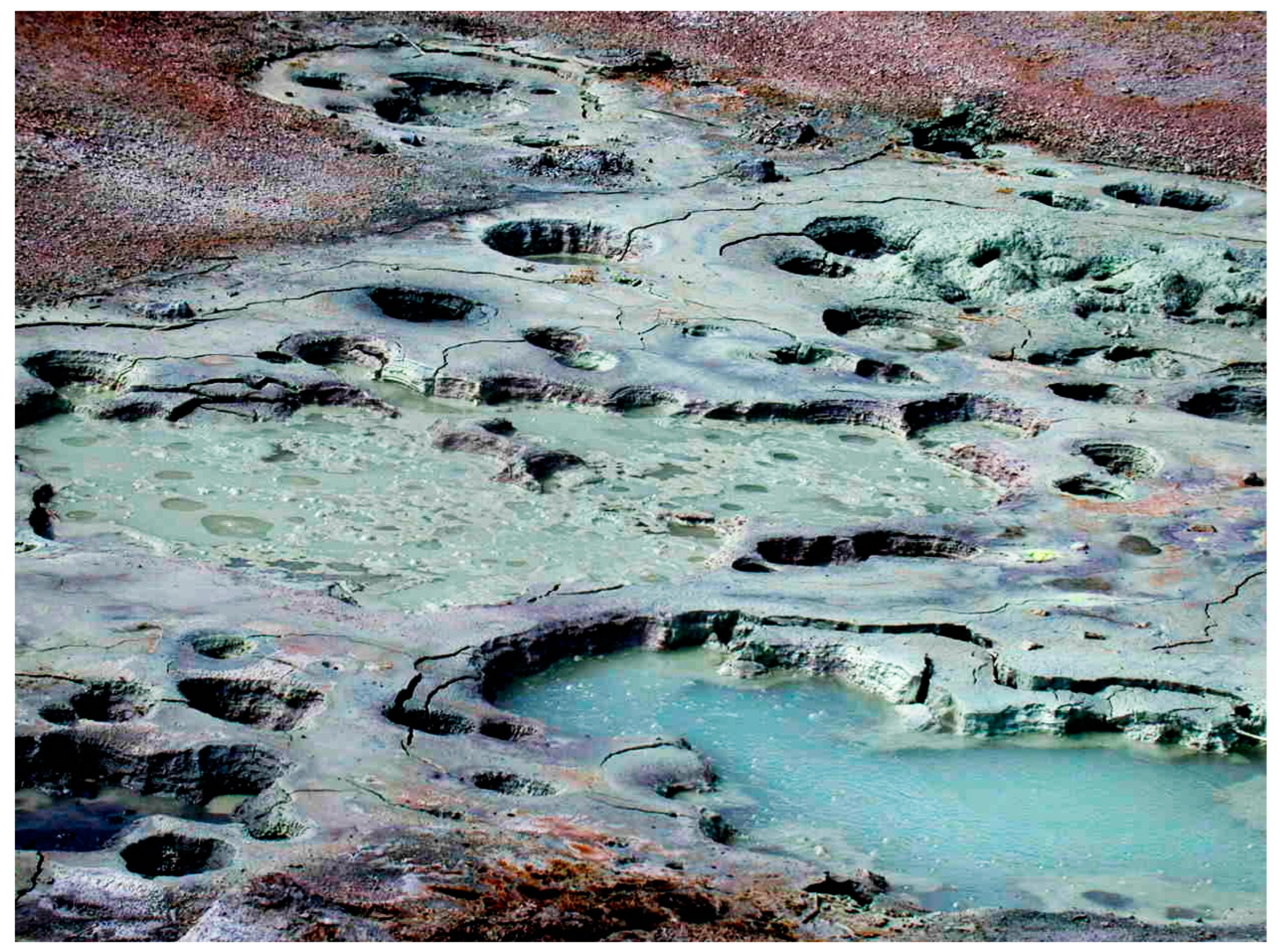This image appears to depict an abstract, colorful landscape, likely an artistic interpretation of geothermal activity, such as that found in Yellowstone National Park. The scene is a chaotic blend of vibrant watercolors, with hues ranging from teal, aqua, and green to pink, purple, red, and orange. The composition is filled with numerous holes and craters, some of which contain bubbling liquids, suggestive of heat emanating from below. This variegated landscape seems to portray the rich mineral tapestry characteristic of geothermal areas. The soil and water display unusual colors, with greens dominating large sections and transitioning to whites and reds at the periphery. Though the image presents itself with the ambiguity of abstract art, its detailed portrayal evokes the dynamic and colorful nature of geothermal environments.